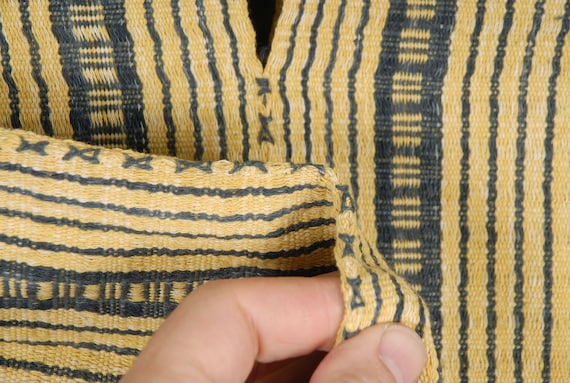The image is a close-up of a light-skinned person's hand holding a small piece of textured fabric between their thumb and pointer finger at the bottom center of the frame. The fabric, which they are feeling to gauge its texture, is primarily a light yellowish color with black lines running vertically. Along the edges of the fabric, there are black patterns resembling hourglass shapes or X's. At the top center of the image, a small black triangle is visible, suggesting the fabric is parting slightly. Flanking this, to the left and right, are larger, ladder-like shapes composed of thick dark gray or black bars running vertically with horizontal bars in between, akin to the steps of a ladder. The fabric might be part of a sleeve edge, and the photo's background shows a larger section of similar fabric.